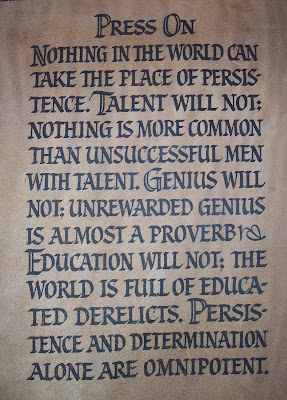This photograph showcases a decorative piece hanging on a wall, illuminated by a gentle wash of natural sunlight streaming in from an unseen source. The artwork appears to be printed on either parchment or a wooden surface, lending it a rustic and timeless quality. The text, rendered in a font reminiscent of classical serif styles with elegant flourishes, includes an eye-catching blend of large and small capital letters.

The content of the text is formatted into a neat, justified rectangle, creating a visually balanced block that commands attention. At the top, the words "PRESS ON" are prominently displayed in bold capitals. Below this heading, the philosophical message is laid out over approximately 12 to 15 lines, each letter meticulously capitalized, with the initial letters of the sentences rendered slightly larger.

The inscription reads:

"NOTHING IN THE WORLD CAN TAKE THE PLACE OF PERSISTENCE. TALENT WILL NOT; NOTHING IS MORE COMMON THAN UNSUCCESSFUL MEN WITH TALENT. GENIUS WILL NOT; UNREWARDED GENIUS IS ALMOST A PROVERB. EDUCATION WILL NOT; THE WORLD IS FULL OF EDUCATED DERELICTS. PERSISTENCE AND DETERMINATION ALONE ARE OMNIPOTENT."

Amidst the text, following the word "proverb," a delicate illustration of a twig with a single leaf extending to the right adds a natural touch, symbolizing growth and continuity amidst the powerful words. All these elements come together to make this piece both an inspiration and a visual delight.